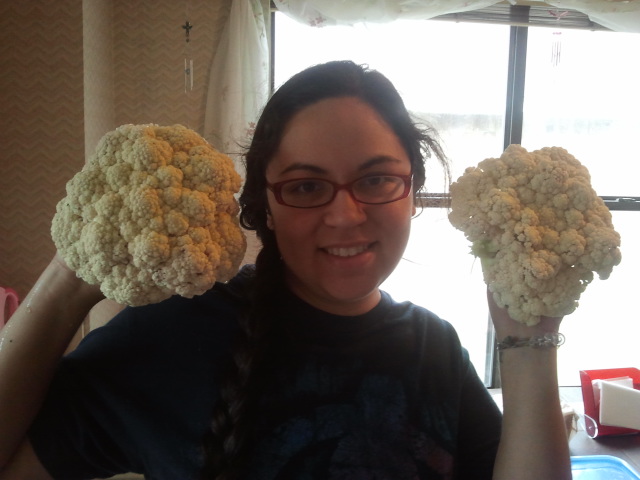A young woman is standing indoors, prominently in the center of her kitchen, posing with a smile. She has dark brown hair pulled back and cascading down her shoulder in a braid, and she's wearing distinctive red-framed glasses. Dressed in a black tank top, the woman holds up two fully bloomed, healthy heads of cauliflower, one in each hand, positioning them beside her head for the camera. Her left arm appears wet, suggesting she might have just washed the vegetables. The background features a large window draped with white curtains and beige-yellow wallpaper, possibly indicating a snowy scene outside. The overall ambiance of the image is warm and inviting, enhanced by the natural light from the window.